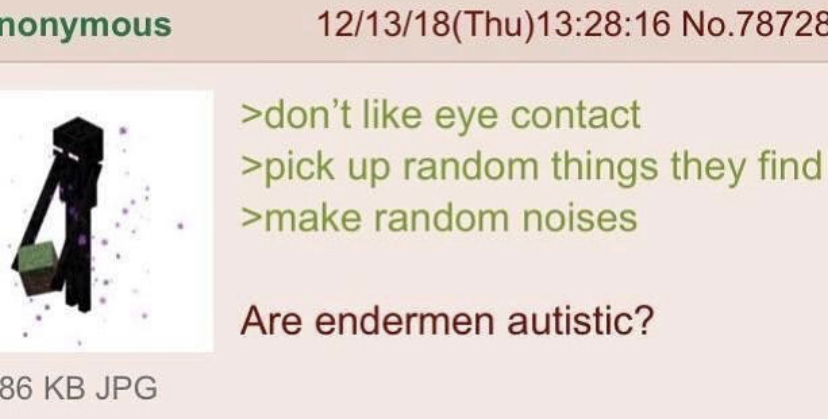The image is a rectangular partial screenshot, possibly from a computer or phone. The background is largely a light pink color, with a darker pink band running across the top. In the top left corner, there is the word "nonymous" in green, although the "A" is cut off. To the right, it displays in red the date "12/13/18" followed by "(Thursday)," the time "13:28:16," and the number "78728." 

Below this header, the lighter pink area contains text in green that reads: "don't like eye contact, pick up random things they find, make random noises." Directly beneath this in red is the question: "Enderman autistic?" 

On the left side of the image, there is a digitally created creature composed of different-sized black boxes, resembling a tall, blocky figure with long limbs. It is holding a small green block, reminiscent of a wooden playing block for children. The background behind the creature is white with some gray speckles. 

In the bottom left corner, partially cut off, is the file size displayed in gray text: "86 KB JPG."